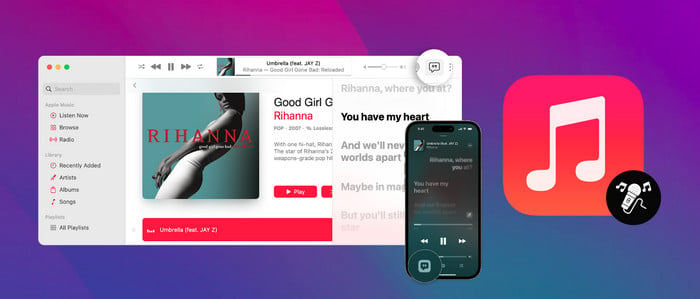The image features a vibrant advertisement for a music application or website, set against a purple background with a pinkish gradient at the top. On the left side, there's a website interface with a photograph of Rihanna dressed in white against a blue backdrop. The text "Good Girl" and "You Have My Heart" are displayed prominently. This white and grey interface includes a list of directories and a currently playing song at the top. Towards the right, there's a smartphone screen displaying the same song interface. To the far right, there's a red square button featuring a white musical note, with a circular black icon beneath it showing a microphone and musical notes. This detailed layout suggests the advertisement is promoting both the song and the app for playing or purchasing it.